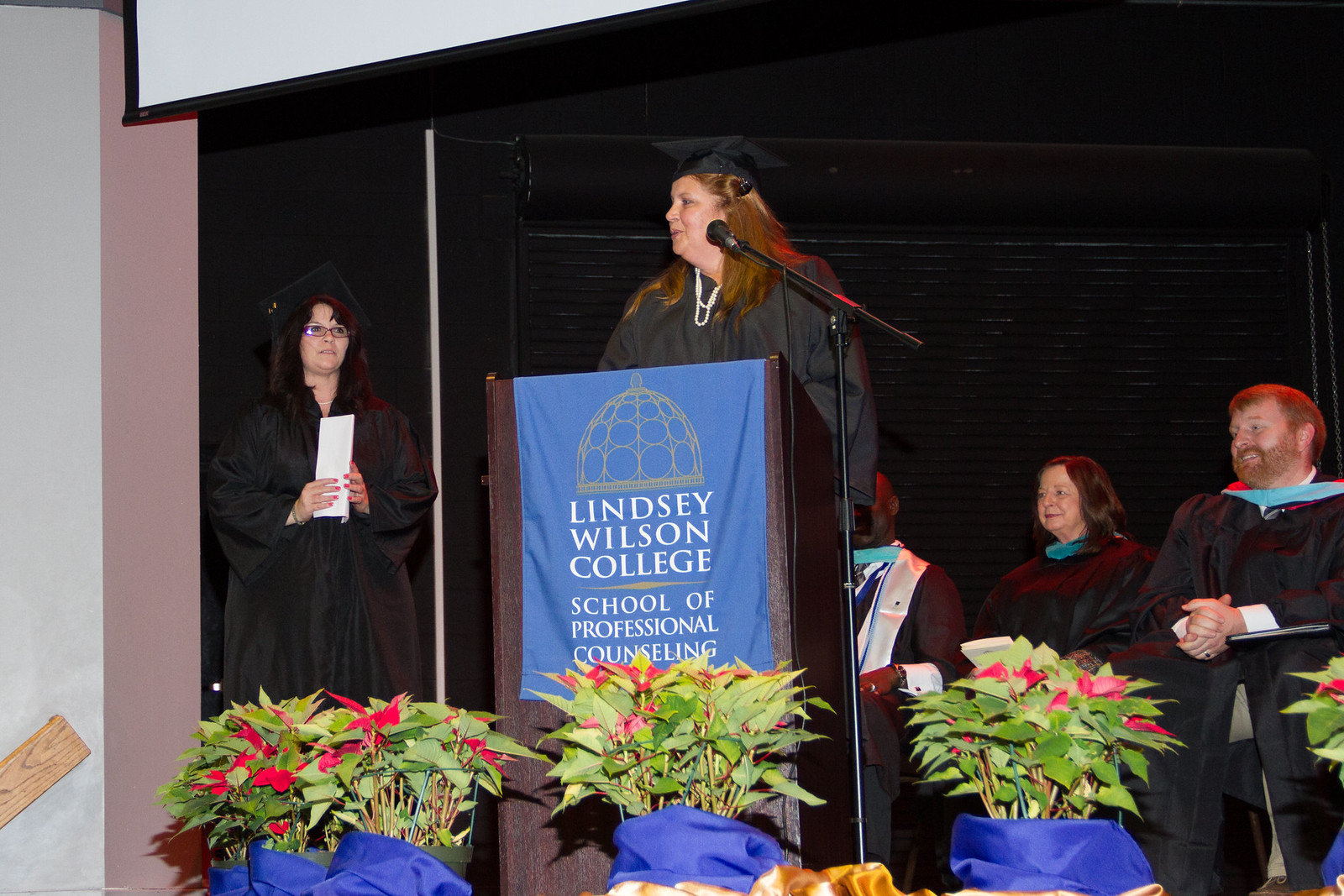This photograph captures a poignant moment at a college graduation ceremony. At the forefront, standing at a podium draped with a blue cloth inscribed with "Lindsay Wilson College, School of Professional Counseling," is a woman with brown hair, appearing to deliver a speech. The podium is decorated with three vibrant floral arrangements, featuring red flower petals, adding a touch of elegance to the scene. Surrounding the woman are four individuals dressed in traditional black graduation gowns with light blue collars peeking through. One of these individuals is positioned to the side, holding a white piece of paper, possibly a speech or a program. The remaining three are seated, attentively facing the audience, presumably proud family members or faculty. The atmosphere is filled with a sense of achievement and anticipation, as the woman at the podium gazes into the distance, encapsulating the milestone moment of her graduation.